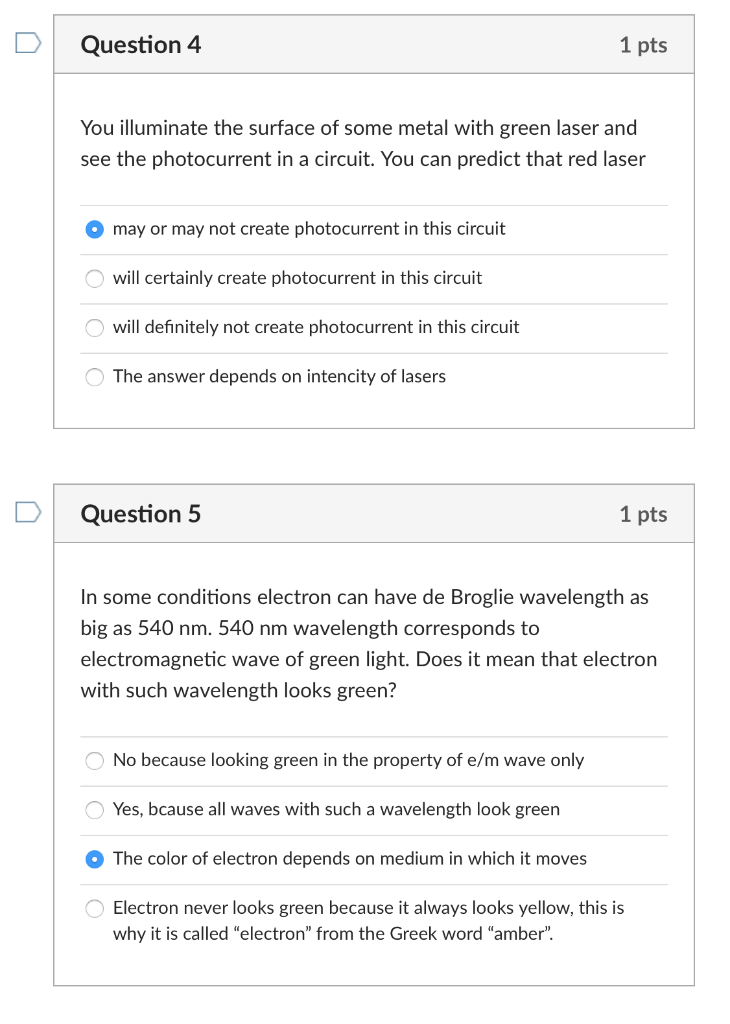**Caption: Physics Exam Question Overview**

The top section of the image features a square highlighted with the prompt: "Question for one point." The question focuses on the photoelectric effect, stating that when a metal surface is illuminated with a green laser, a photocurrent is observed in the circuit. It then speculates about the effects of using a red laser, with the selected answer indicating uncertainty ("may or may not create photocurrent in this circuit"). Below, three options are presented: 
1. It will certainly create photocurrent in the circuit.
2. It will definitely not create photocurrent in the circuit.
3. The answer depends on the intensity of the lasers.

Further down, "Question 5 for one point" introduces a scenario involving an electron with a de Broglie wavelength of 540 nanometers, a wavelength corresponding to green light in the electromagnetic spectrum. The question asks if this means the electron appears green. The selected answer, "the color of the electron depends on the medium in which it moves," is contrasted with other choices:
1. No, because looking green is the property of electromagnetic waves only.
2. Yes, because all waves with such a wavelength look green.
3. The electron never looks green because it always looks yellow since the term electron comes from the Greek word for amber.

The image captures an educational snippet designed to test students' understanding of photoelectric effects and wave-particle duality.